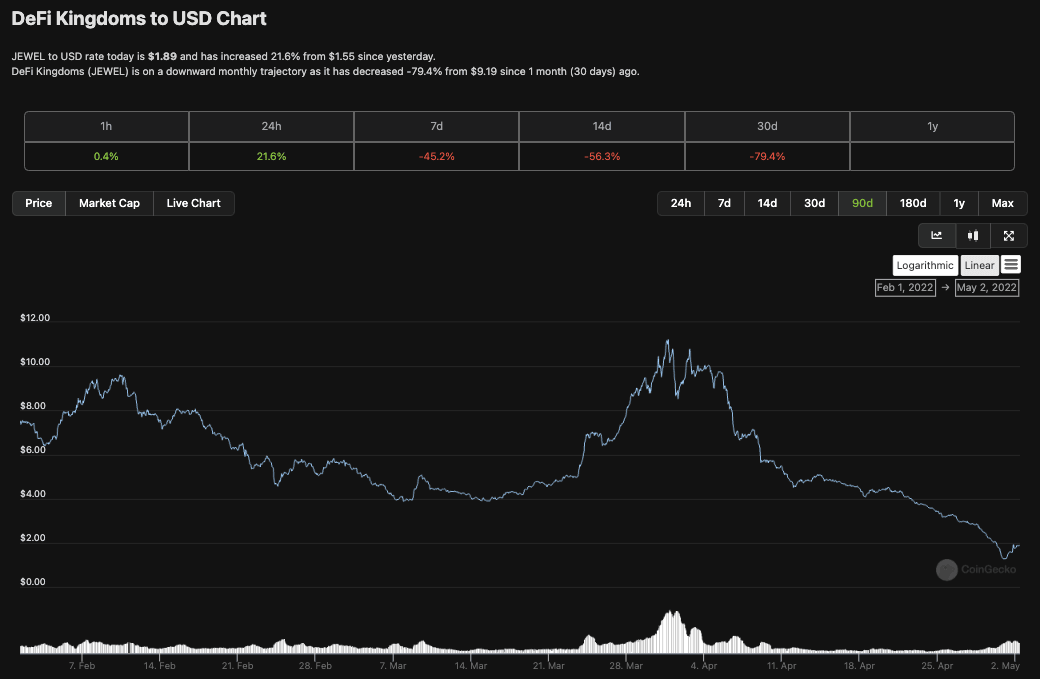A screenshot of a computer screen displaying a cryptocurrency pricing chart on a black background. The chart, titled "DEFI Kingdoms to USD Chart," in white text at the top left corner, tracks the value of "Jewel" in USD. Below the title, it states that the "Jewel to USD rate today is $1.89," indicating a 21.6% increase from the previous day's value of $1.55. Further details mention that DEFI Kingdoms (Jewel) is experiencing a downward trend, having decreased by 79.4% from $9.19 one month ago.

The chart features six columns, each representing different time frames: one hour, 24 hours, seven days, 14 days, 30 days, and one year. The percentage changes in Jewel's price for each timeframe are displayed, with green text for positive changes and red text for negative changes. Specifically, the changes are: 
- One hour: +0.4% (green)
- 24 hours: +21.6% (green)
- Seven days: -45.2% (red)
- 14 days: -56.3% (red)
- 30 days: -79.4% (red)
- One year: No data provided

Below the chart, in bright white text, are options for "Price," "Market Cap," and "Live Chart." Toward the right side of the screen, time frame options for graph visualization include "24 hours," "7 days," "14 days," "30 days," "90 days" (in green), "180 days," "1 year," and "Max" in white text.

A graph on the right side of the screen plots the Jewel price on the y-axis, ranging from $0 to $12, while the x-axis spans from February 1, 2022, to May 2, 2022, displaying two fluctuating lines indicating the price movements over this period.